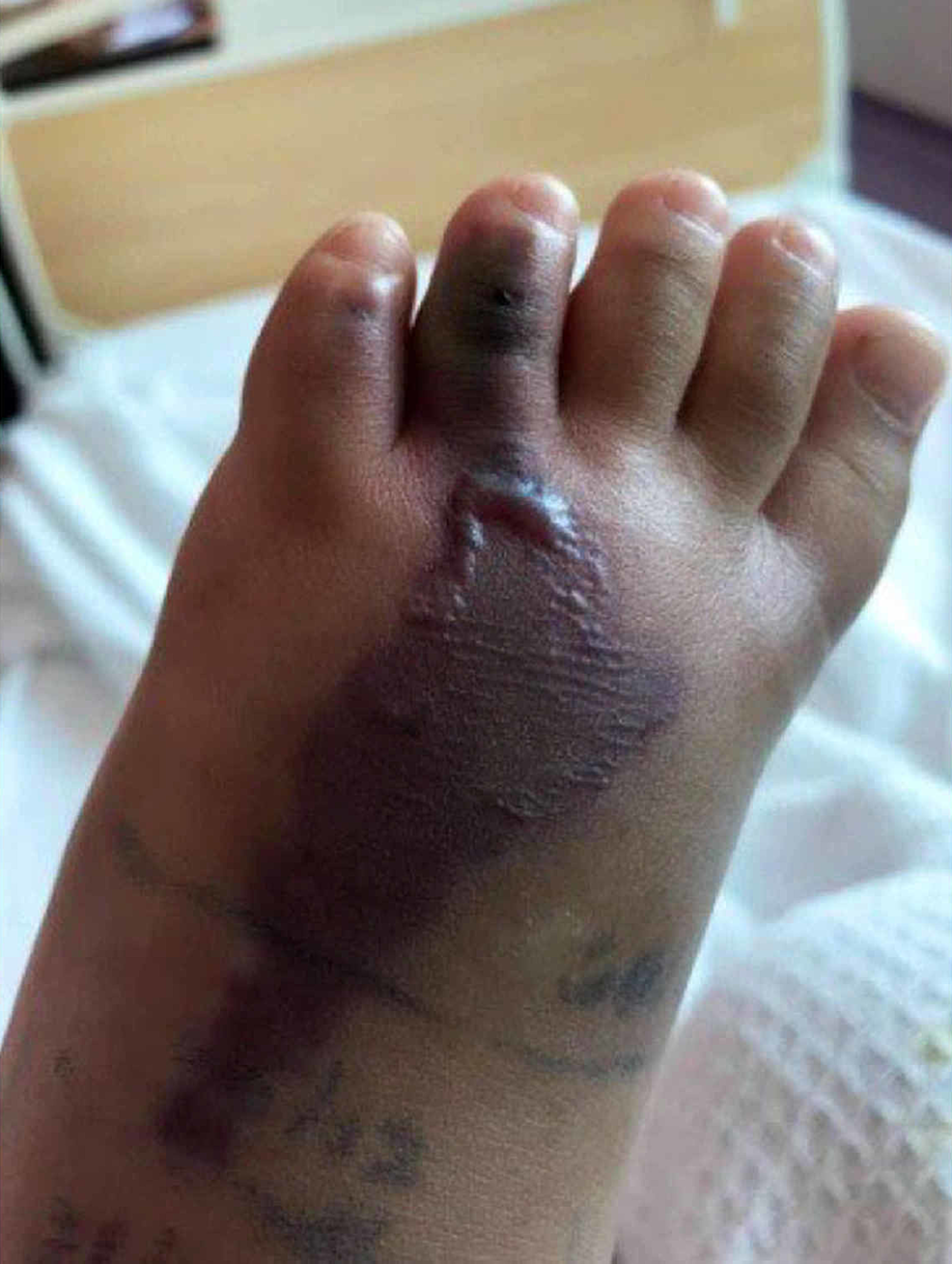The image depicts a close-up of a severely swollen left foot, belonging to what appears to be a young African-American child, possibly between 11 to 12 years old. The foot is positioned over a hospital bed, identifiable by the blurred white bedding and nearby medical surroundings. The skin is dark brown with a strikingly large, darker rash resembling the shape of South America, situated prominently on the top of the foot, extending upwards beneath the toes. The rash appears to have a blister near the index toe. The toenails are neatly trimmed, though the toes are also swollen. Handwritten surgical markings are faint yet visible on the foot, suggesting preparation for an upcoming procedure to address the condition. The overall scene underscores a sense of medical urgency and care, as the child's foot, marked by varying degrees of swelling and discoloration, awaits treatment.